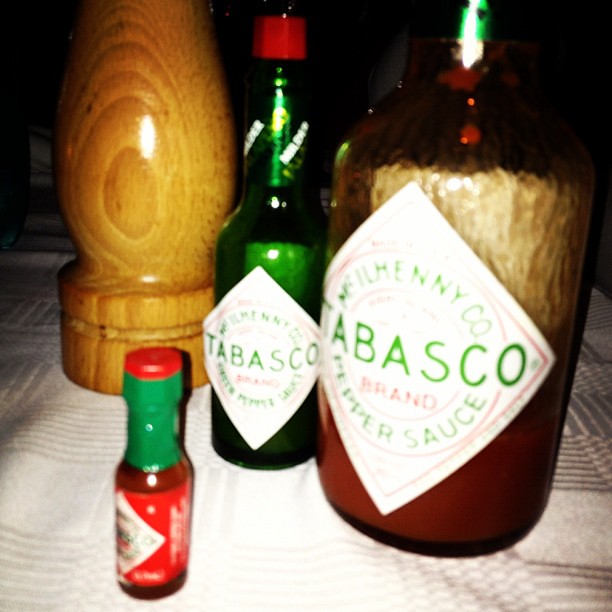In this detailed up-close photograph, taken with a flash in a dark room, the focus is on an assortment of Tabasco bottles arranged on a luxurious, white tablecloth featuring light brown stripes. The central object is a medium-sized green glass bottle of Tabasco sauce with a red cap and a distinctive red and white label featuring "MCILHENNY Co." in green text and a red diamond logo. To its left is a tiny one-use bottle of Tabasco with a red label, red liquid, a green neck, and a red cap. Behind and slightly to the left of these two bottles is the bottom half of a polished brown wooden container, possibly a pepper grinder with a teardrop shape, assumed to be made of dark walnut wood. A larger brown bottle, also with a Tabasco label similar to the others, stands to the right of the green bottle, partially out of view. The flash of the camera creates a shiny reflection on the wooden container and the glass bottles, while the background remains obscured, giving the scene a dramatic and intimate ambiance.